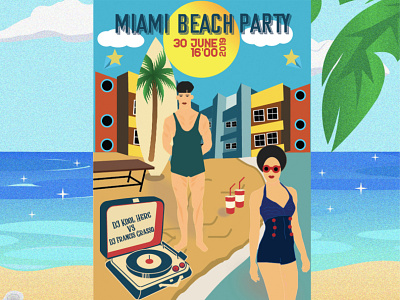The flyer for the "Miami Beach Party" event is set against a picturesque backdrop of a vibrant blue sky with scattered clouds, glistening blue and teal waters, and golden sand. Dominating the center is text announcing the party, with a large, stylized sun graphic overhead that contains the event details: "30 June 2018 at 1600." 

In the foreground, a vintage record player is positioned on the sandy beach, its black top and red interior showcasing a small vinyl record with the tone arm poised to play. Standing by the record player is a figure in a light blue, old-timey one-piece swimsuit that resembles a romper, characterized by its sleeveless design, low neckline, and short shorts. This person, with light skin and dark hair, is complemented by a woman beside him, similarly dressed in a distinct two-tone blue swimsuit adorned with six red buttons on each side. She sports red sunglasses, red lips, and a hat, her light skin and brown hair adding to the vintage aesthetic.

To the right of the couple, Miami’s skyline is visible with multicolored buildings in hues of yellow, pinkish-red, blue, and teal. The beach scene is accentuated by a couple of drinks nestled in the sand, a surfboard featuring a palm tree design, and additional palm fronds. The whole setting is bathed in the nostalgic charm of 1920s beachwear, encapsulating the festive and retro spirit of the Miami Beach Party invitation.